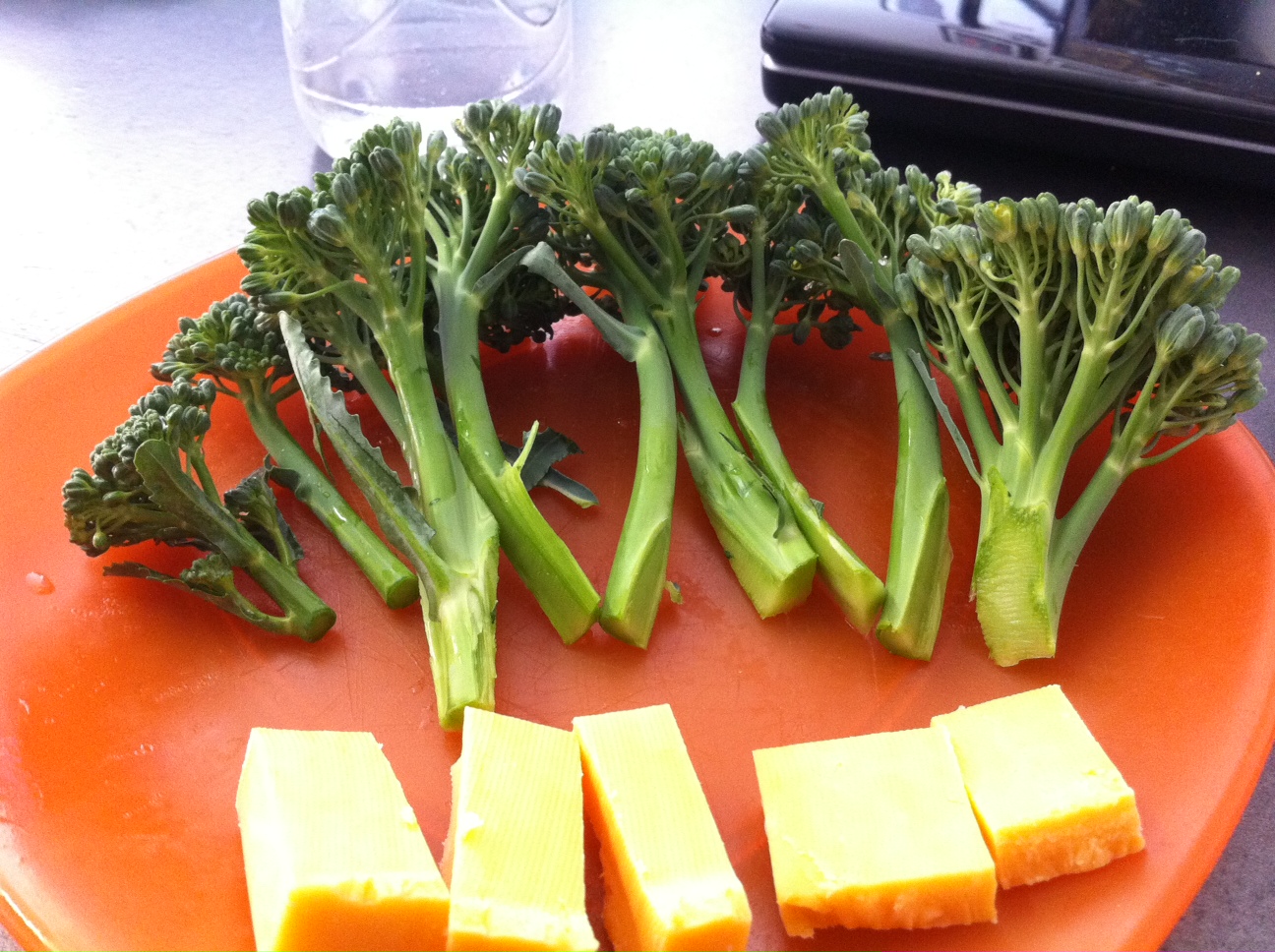This image captures a vibrant, round orange plate, likely made of plastic or ceramic, serving a healthy snack. Dominating the plate are several stalks of fresh broccoli arranged in a slight arc at the top. The broccoli, possibly broccolini, showcases vibrant green stems with darker blue-green florets, some still adorned with leaves. Below the broccoli, there are five pieces of cut cheese, presumably Colby Jack or cheddar. The cheese varies in shape, with two pieces cut into squares and three into rectangles, displaying a gradient of color from yellow-orange to almost white due to the lighting. The detailed arrangement reveals the largest pieces on the left gradually getting smaller to the right.

In the background, occupying the top left corner of the frame, is a partially filled clear glass or water bottle. This item extends off the page, catching some reflective light. To the top right of the image, there’s a hint of an enigmatic rectangular black object with reflective properties, possibly office equipment. The entire setup is situated on what appears to be a light gray or silver surface, dappled with bright light from the left side, rendering a clean and organized presentation of a nutritious and appealing snack.